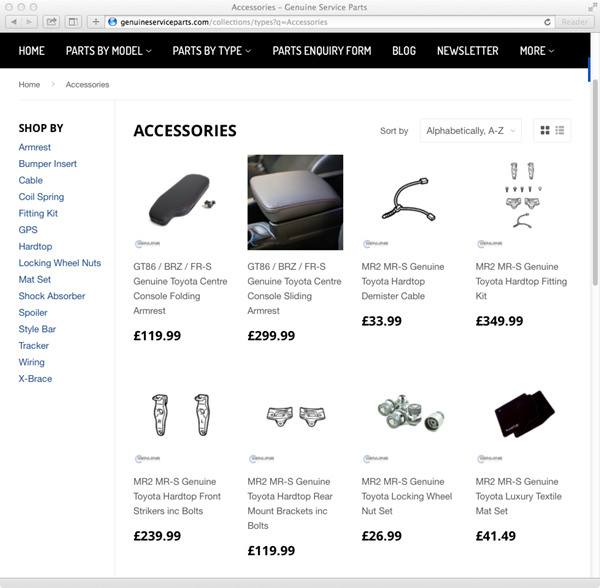**Caption:**

This post features a screenshot of a vintage website interface, seemingly captured from an old Mac computer, recognizable by the traditional layout and distinctive icons at the top left corner—red for closing, and additional options for website interactions. The website, genuine-services-parts.com, as indicated by the search results at the top, has a navigation menu with sections like Home, Parts by Model, Parts by Type, Parts in Query Form, Blog, Newsletter, and More. The screenshot specifically displays the 'Home' page, with a sub-menu leading to a more detailed 'Accessories' section. Here, various Toyota accessories are listed, such as the Genuine Toyota Central Console Folding, Genuine Toyota Central Console Sliding, and Genuine Toyota Hardtop Demonstrate Cable. The abundance of Toyota-related accessories suggests that a Toyota model was likely specified earlier. This detailed navigation offers a plethora of options for Toyota vehicle enthusiasts.